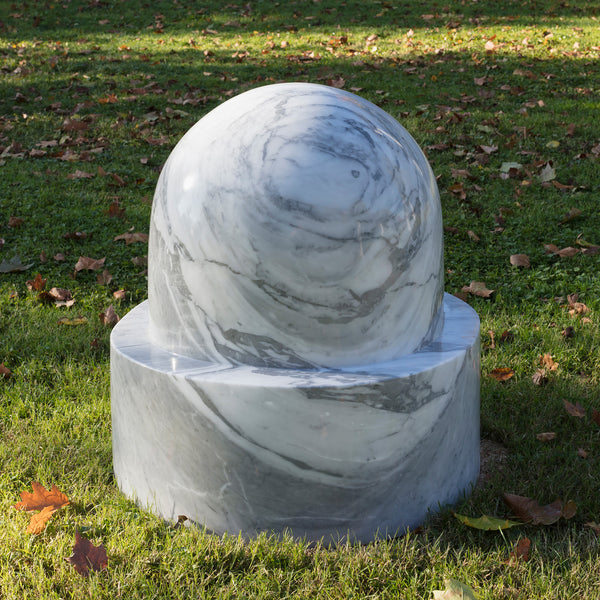This image captures a marble statue in an outdoor park setting. The statue, composed of a marble with a milky tone and a swirling cloud-like texture, features an abstract geometric design. The top part of the statue is a spherical shape, seamlessly fused into a circular base beneath it, both sharing a distinctive pattern of gray and black splotches reminiscent of water. The statue is positioned on a grassy field strewn with dead leaves in shades of brown and orange, indicating the autumn season. Shadows from objects outside the frame partially cover the grass and statue, suggesting it is late afternoon with the warm light of the setting sun illuminating the scene.